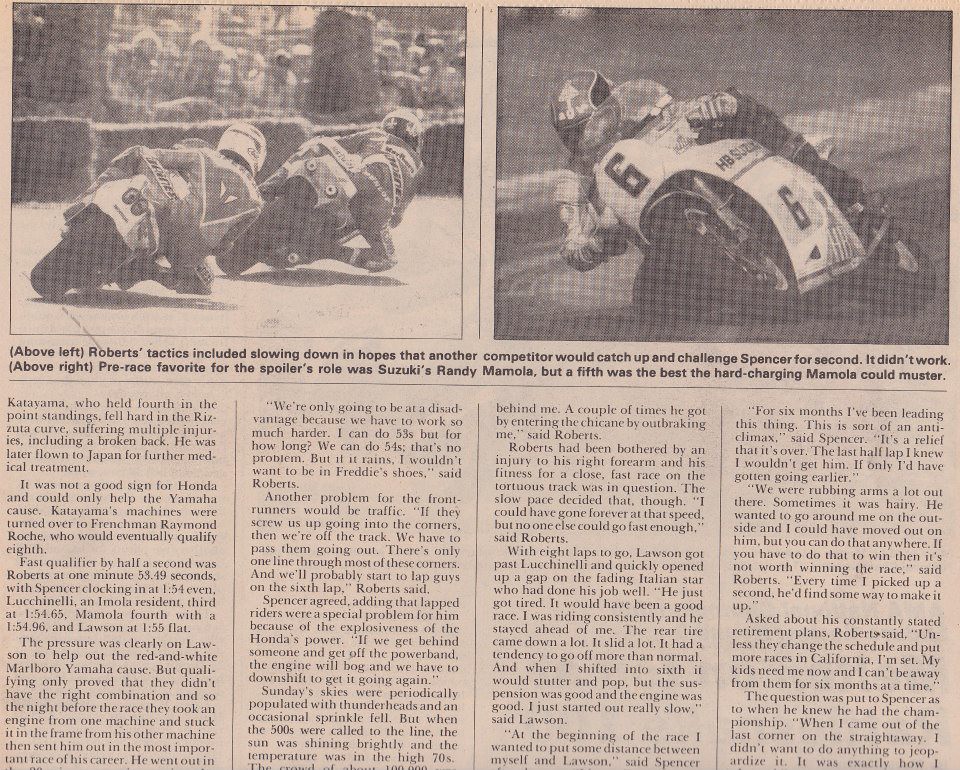The image is a single object that appears to be a page from an old, yellowed newspaper, predominantly off-white with black and various shades of gray. At the top of the page, there are two black-and-white photographs of motorcycle racers. The photo on the left shows two men racing on a track, leaning so far to their right that their knees are nearly scraping the ground. Straw bales or barriers are visible in front of them, and a stadium with blurred spectators lines the background. The photo on the right captures a lone racer on a white motorcycle marked with the number six, his elbow almost touching the ground due to his extreme lean. Below these images, captions read: "above left, Roberts' tactics included slowing down in hopes that another competitor would catch up and challenge Spencer for second. It didn't work." and "above right, pre-race favorite for the spoiler's role was Suzuki's Randy Mamola, but a fifth was the best the hard-charging Mamola could muster." The main article text occupies the lower part of the page, divided into about four sections. The entire layout and styling emphasize the dated and classic nature of the newspaper page.